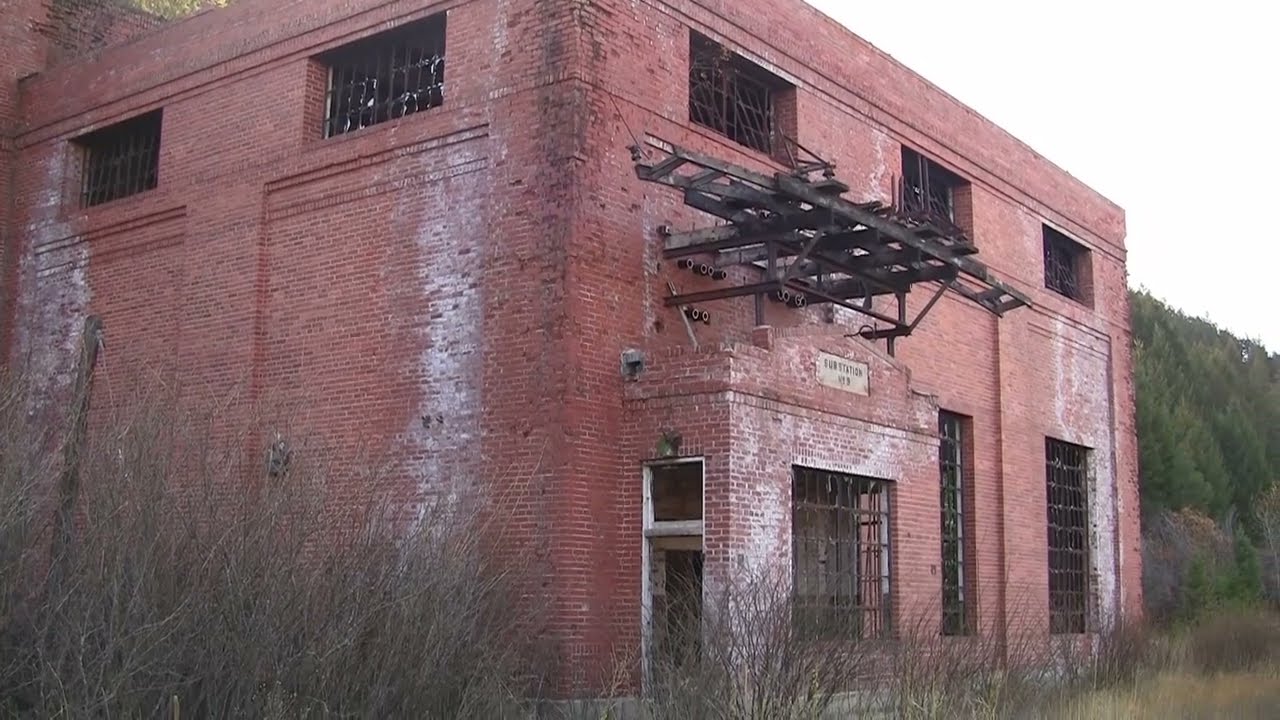The image depicts an abandoned, square-shaped old factory or warehouse constructed from red brick, though the bricks are somewhat faded in sections. The windows, all of which are broken or missing, revealing only the dilapidated frames, are reinforced with rusted black security bars. These windows are predominantly rectangular with square ones higher up on the building. Above the front entrance, there is a dilapidated, junk-like structure resembling an awning or a black steel ladder. The bricks are marked with white streaks from mineral deposits due to water damage. The building features unreadable graffiti on the front door and stands amid overgrown dry brush, grass, and trees, which are dense around the sides and in the distance. The overall scene suggests a forlorn and neglected piece of industrial history overtaken by nature.